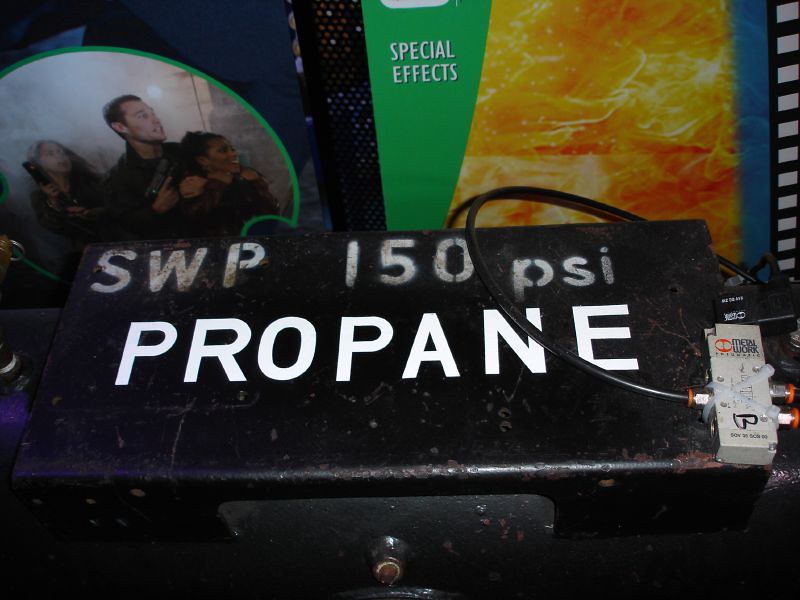The image depicts an intriguing and somewhat complex scene centered around a black metal box labelled with "SWP 150 PSI" and "propane" in bright white letters. Atop this box, there's a cord connecting to a grey hub, emphasizing its electronic or mechanical nature. On the right side of the black box, there's a switch with two red buttons, bearing the word "metal work" and a "B" marked in black. Behind the black box are advertisements, seemingly movie or magazine covers. One advertisement prominently features flames and the phrase "special effects," while the other showcases three characters: a man holding a gun and one of two women hostage. The image is well-lit, providing clear visibility of all elements and creating a vivid, detailed scene.